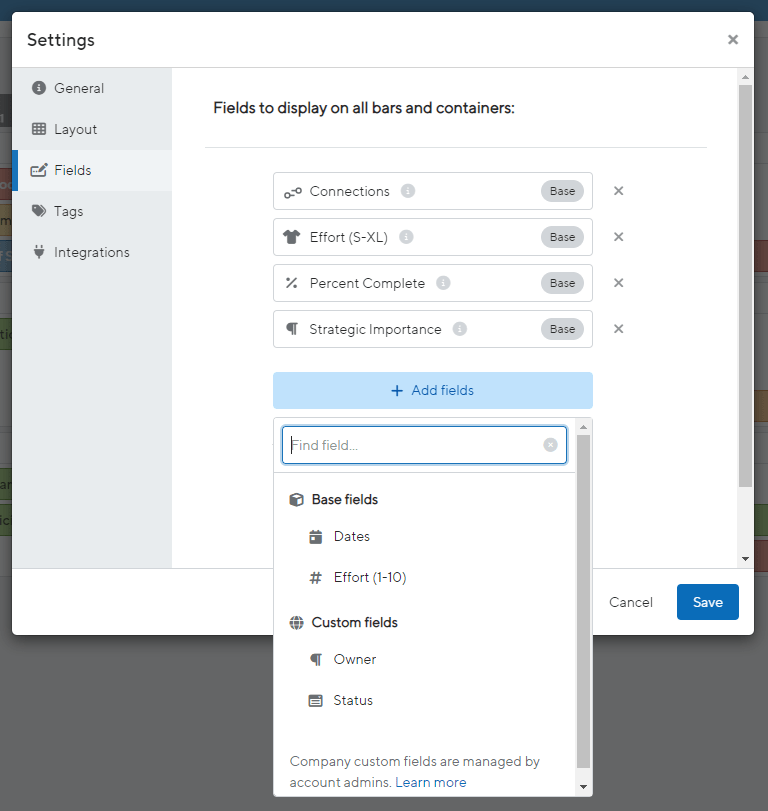**Detailed Caption:**

The image depicts a screenshot of the settings page of an application or software interface on a computer or device. At the top of the interface, the heading "Settings" is prominently displayed. Along the left-hand side of the page, a vertical navigation menu lists several options: "General," "Layout," "Fields," "Tags," and "Integrations." The option labeled "Fields" is highlighted with a blue line, indicating it is the current selection.

In the central portion of the screen, under the heading "Fields to display on all bars and containers," various field categories are listed in sectioned rows. These include:

- "Connections"
- "Base"
- "Effort"
- "S to XL"
- "Base"
- "Percent Complete" (with an associated percentage)
- "Base"
- "Strategic Importance"
- "Base"

A "+" icon next to "Add Fields" is visible, along with an adjacent "Find Field" option. Further down, the list includes default field categories such as "Base Fields," "Dates," "Effort," "1 to 10," "Custom Fields," "Owner," and "Status."

In the bottom right-hand corner of the interface, a prominent blue "Save" button is available for the user to confirm any changes made on the settings page.